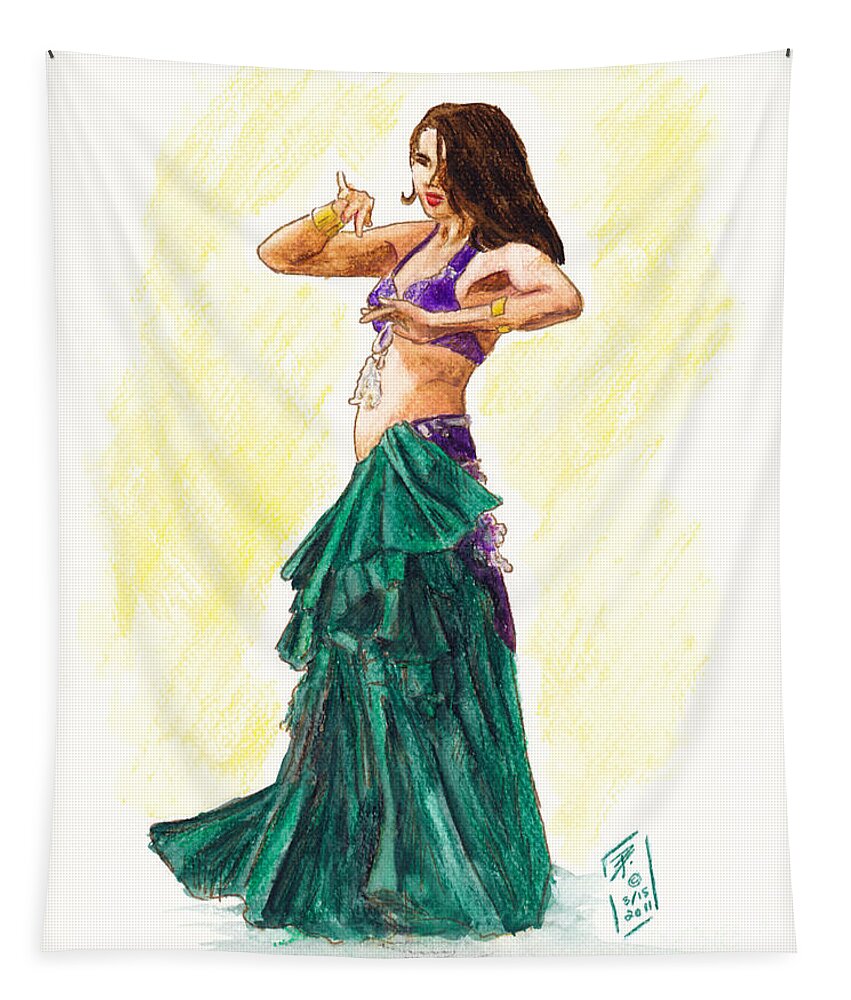This detailed painting on a white sheet, pinned at the corners, vividly portrays a belly dancer in mid-dance. The woman has long brown hair that partly covers one eye, and she's adorned with a striking purple bra and complemented with golden jewelry around her wrists. Her flowing green skirt, which has purple undertones on the backside, extends to the floor with ruffles adding a sense of movement. Her midriff is bare, enhancing the authenticity of her belly dancer appearance. The background features subtle yellow paint, adding contrast to the white sheet. Her arms are elegantly lifted in a classic dance gesture, showcasing her finger movements. Red lipstick and detailed facial makeup complete her look. The artwork is signed in a foreign script with the date "3-15-2011" in the bottom right corner, anchoring the piece with a personal touch.